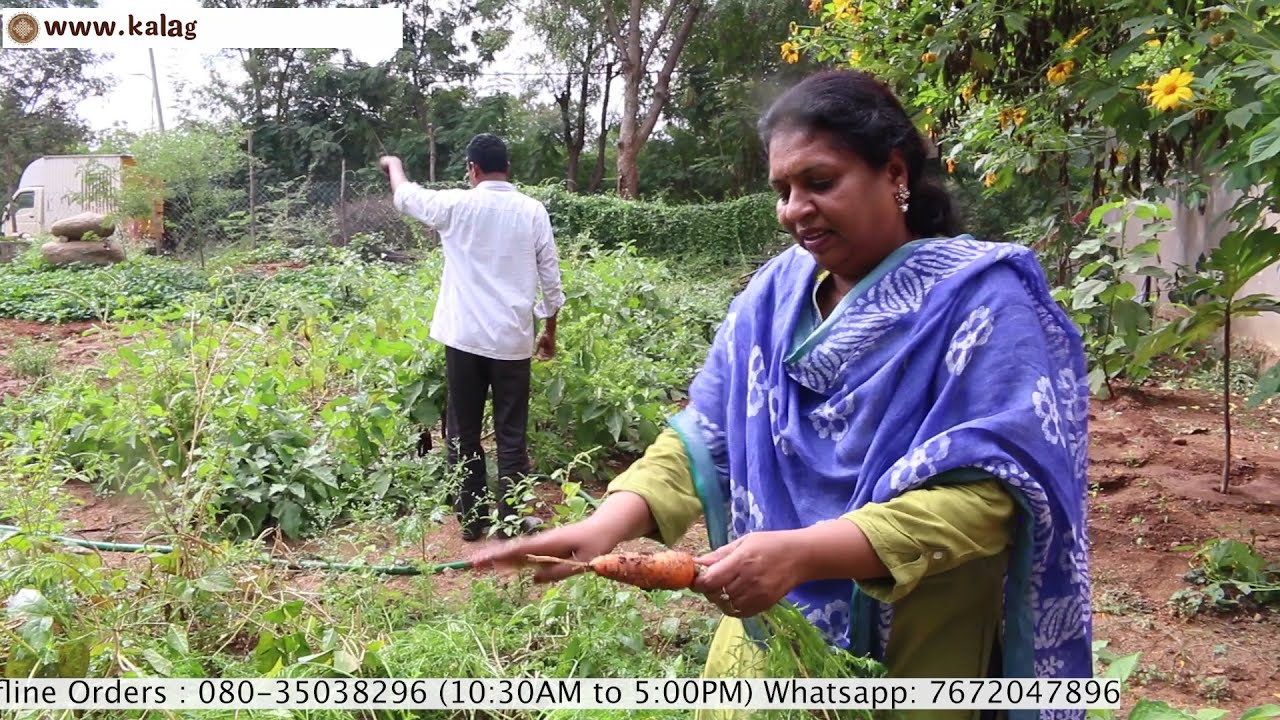In this vibrant outdoor setting, the photograph depicts a diverse garden scene bustling with life. At the heart of the image is a woman of East Indian descent, showcasing her long dark hair and caramel-colored skin. She is wearing a long olive-green shirt underneath a distinctive purple poncho adorned with leafy designs and flowers. Draped over her shoulders and arms is a blue and white scarf. Elegant pearl earrings dangle from her ears as she proudly holds a freshly harvested carrot, still dusted with soil, in her left hand.

Behind her stands a man with short black hair, dressed in a white button-down collared shirt and black pants. His back is turned, and he appears engaged in tending to the garden, pointing towards something in the foreground. The setting is lush with greenery, featuring a variety of plants and trees, including sunflower-like blooms. 

The background extends to reveal a white box truck positioned in the top left corner, and the entire scene is bathed in the daylight. Superimposed text in the upper left corner reads "www.KLAG" in brown letters, and additional text at the bottom of the image provides contact information, including a phone number and WhatsApp contact available between 10:30 a.m. and 5:00 p.m. The photograph captures a picturesque moment of communal gardening and outdoor activity, rich in texture and vibrant colors.